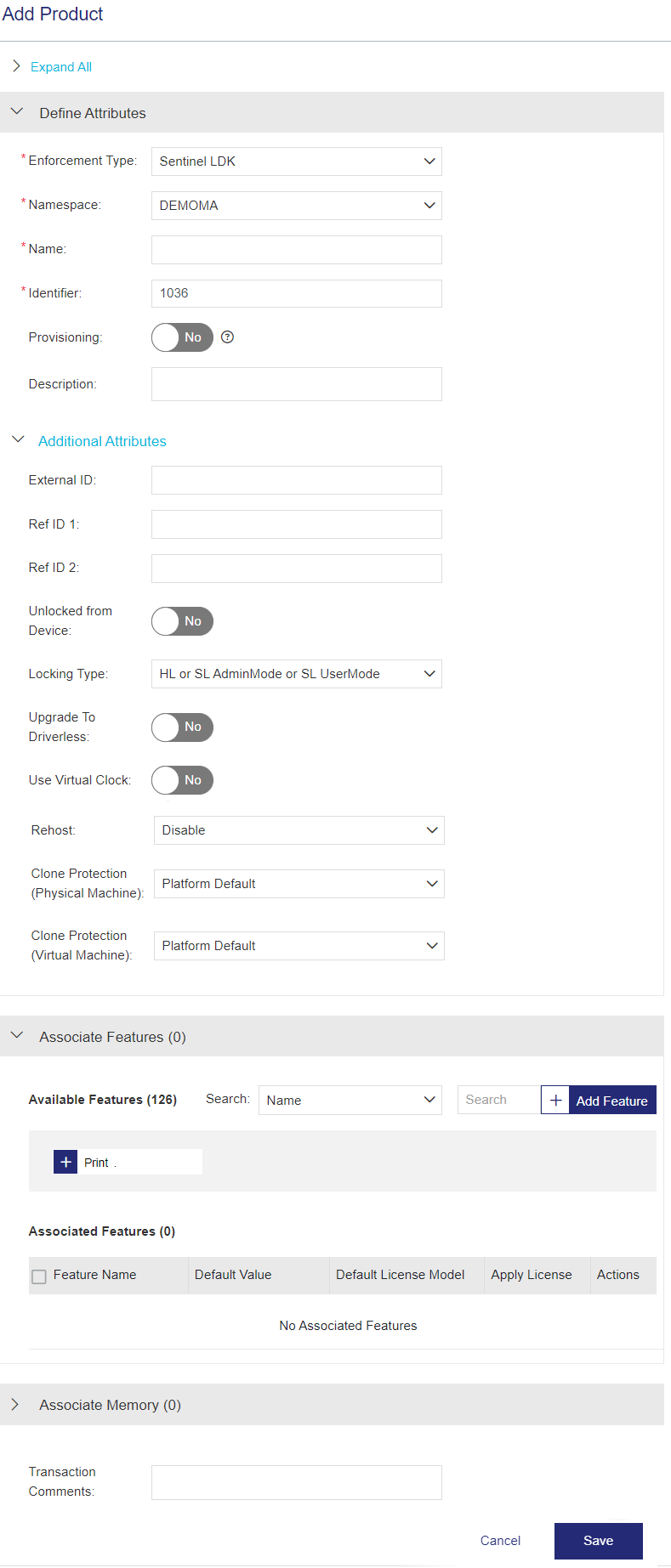This image depicts a zoomed-out view of a webpage, specifically a user interface designed for adding a product. The top of the page prominently displays the heading "Add Product." Directly beneath this heading is a section of light blue text. Following this, the interface transitions to a gray background area which includes a title and three fields of information for the user to fill out.

Continuing down the page, there is a segment with a light blue title accompanied by three additional information fields. Below this section, there is a toggle button, which allows the user to select another option. The category names are aligned on the left side of the interface for easy reference.

The middle portion of the page features two more toggle buttons followed by two fields for further information input. This pattern of alternating backgrounds—between gray and white—with fields to fill out continues throughout the interface.

Towards the bottom of the page, there is a concluding gray background section with additional fields for information input. The overall background of the interface is predominantly white, with light gray sections highlighting specific titles across the width of the page.

Finally, at the very bottom of the interface, there are two options: a "Cancel" option and a dark blue button, which, though small in size, is labeled "Save." This completes the structure of the image.